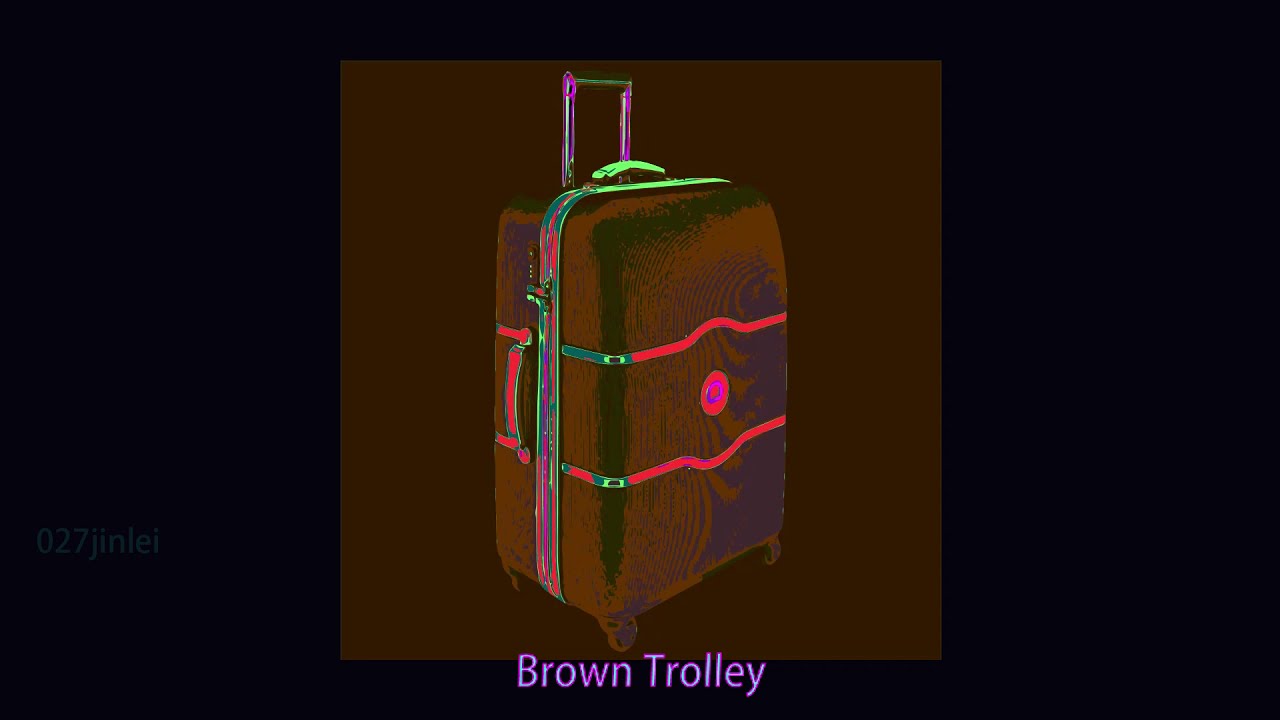The image features a computer-generated, vertically-oriented suitcase, described as a "brown trolley" in purple text at the bottom. The suitcase itself is primarily a brown, hard shell design with a distinctive tilt, providing a head-on view of one of its angles while remaining centered in the image. It boasts neon accents—red, green, purple, and pink—forming lines across its surface. The handle, extended in an upright position, also exhibits purple and green hues with a metallic silver finish. In addition to the main handle, a secondary handle is visible on the left side. The suitcase features a circular logo placed between two red lines. The entire image is wrapped in a brown background, set against a broader black backdrop, evoking a vibrant, club-like aesthetic with its neon lights, suggesting a bold, modern artistic style. The suitcase is depicted with wheels, emphasizing its practical, rollable design.